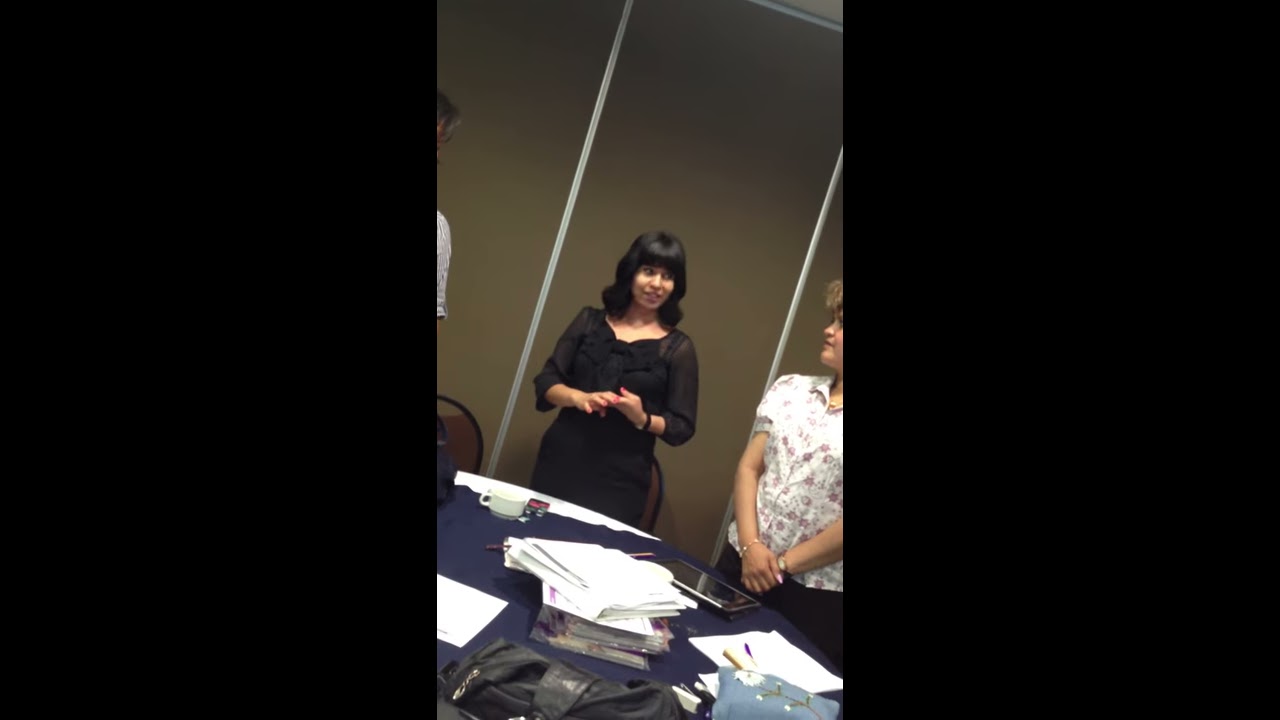In this image, a woman with dark black, wavy hair, dressed in a black outfit, is standing in a meeting room. She appears focused as she looks to her left, engaging with another woman in a white top adorned with floral prints. Both women have pink fingernails and wear watches on their left wrists. To the left of the woman in the white top, there is a man with gray and black hair, wearing a gray shirt. They are all gathered around a table covered with various items, including a tablet, a significant stack of papers, yellow pencils, blue pens, a black bag, and a light blue bag. The table is draped with a blue cloth. The background features a brown wall with vertical gray metal bars and several brown-colored banquet chairs with black frames. The scene suggests a busy and collaborative meeting in a modern office environment.